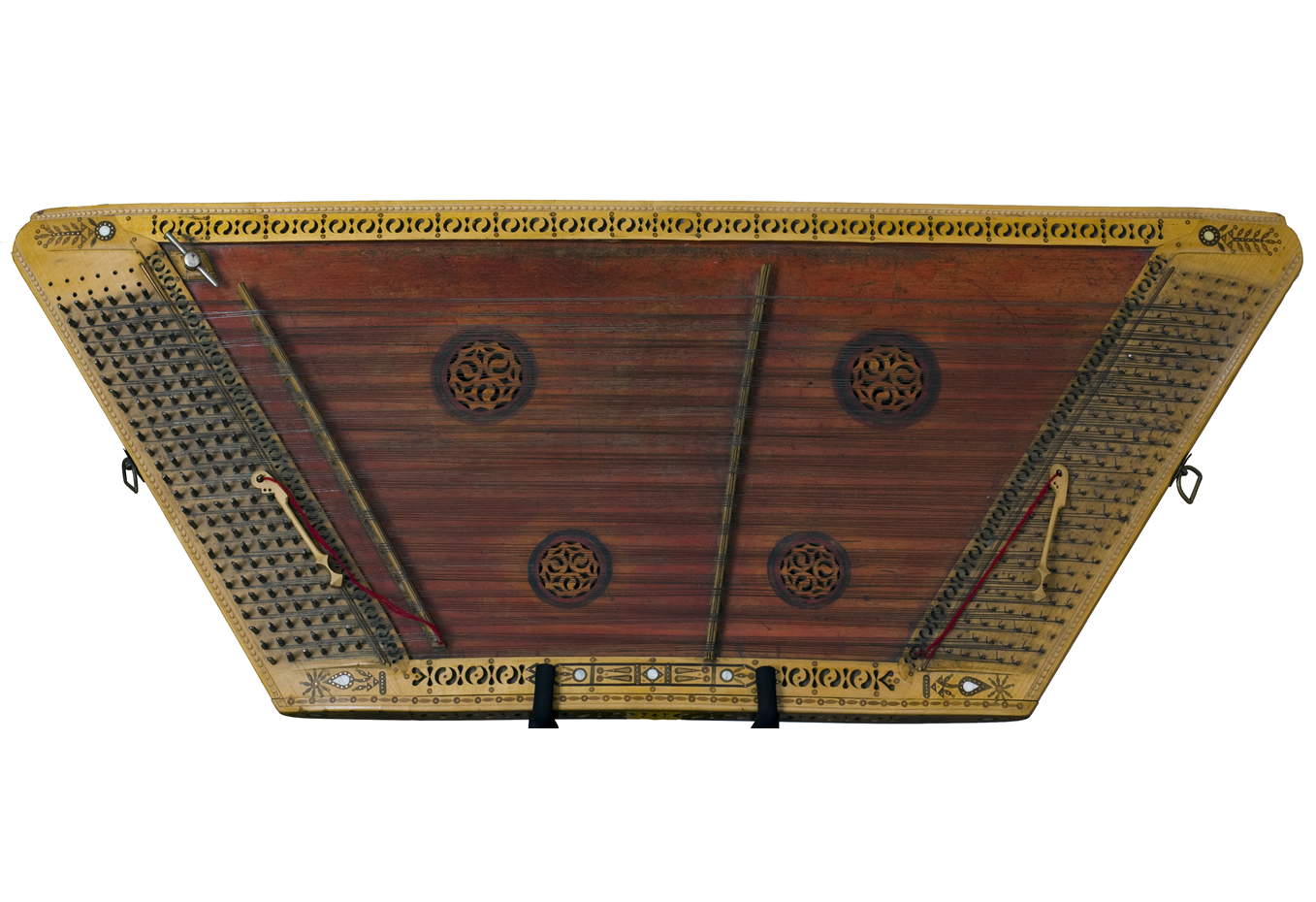In this image, there is a single object positioned at an angle against a white background, ensuring no distractions from its detailed structure. The object resembles a lid, likely not attached to anything, supported by the presence of small metal clasps on both its left and right edges, which presumably serve to secure it when closed. The item has a square-like, almost rectangular shape, showcasing meticulous craftsmanship that hints at an older era.

The outer border of the object is adorned with a gold pattern featuring small O-shaped designs. Moving inward, the interior border transitions to a light brown tone before the center reveals a rich, dark brown wood. This wood section is detailed with horizontal grain lines interspersed with four circular decorations—two at the top and two at the bottom. Each circle has intricate gold designs, possibly reminiscent of sun symbols. Rounding off the details, at the bottom of the object, there are two black tabs, and a red string is also visible, adding a final touch of color to this unique piece.